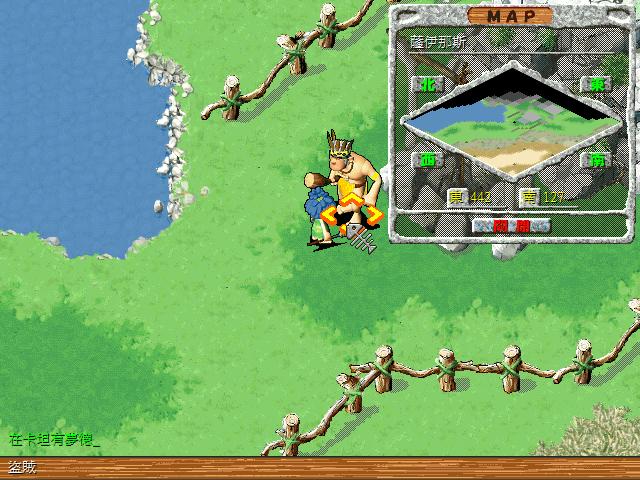This image is a screenshot from an older video game, evident from its poor-quality graphics. Dominating the center of the image is a character who appears to be walking, carrying flowers in one hand and fish bones in the other. The character is dressed in a manner that suggests a historical or indigenous theme, possibly with feathers on their head. The scene is set on a grassy knoll with patches of differently shaded green grass. Logs tied together with twine form crude fences on both the upper and lower borders of the scene. Off in the upper left-hand corner, there's a pool of water surrounded by rocks. 

The game interface is visible as well; in the upper right-hand corner, there's a section labeled "Map" showing a zoomed-in diamond-shaped view of the game's terrain. The area is populated with various words and numbers - 442 and 127 - primarily in an Asian script, which also appears in a watermark located at the bottom right-hand corner of the image. This watermark further implies non-English origins of the game. The image, displaying a combination of textual and visual elements suggests the screenshot might be tracking scores and other in-game statistics.